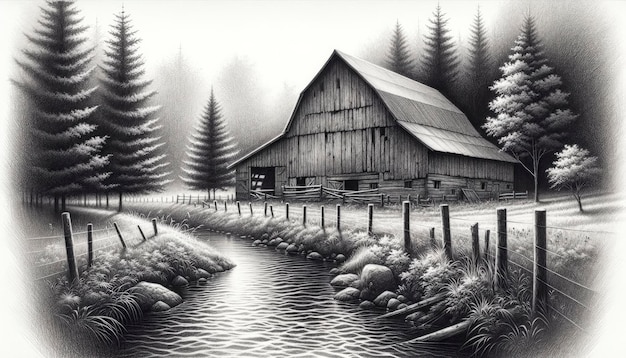This black and white illustration, possibly handmade or computer-generated, depicts an old, weathered wooden barn next to a gentle, narrow creek. The scene is framed with a vignette-like halo that fades into white, enhancing the focus on the barn and its surroundings. Positioned horizontally, the drawing features the barn bordered by a rustic wooden fence interlaced with barbed wire, ensuring it blends seamlessly into the serene, misty woodland backdrop. The woods are populated by evergreen pine trees and a few deciduous trees, some of which are lightly frosted, suggesting a wintry atmosphere, though the running creek indicates it isn't too cold. The barn itself appears neglected and aged, with worn wood facades and covered entrances where doors or windows once were. Towering trees and scattered shrubs give depth to the tranquil, picturesque setting, capturing a quiet moment in what seems to be a historical, rural farmstead.